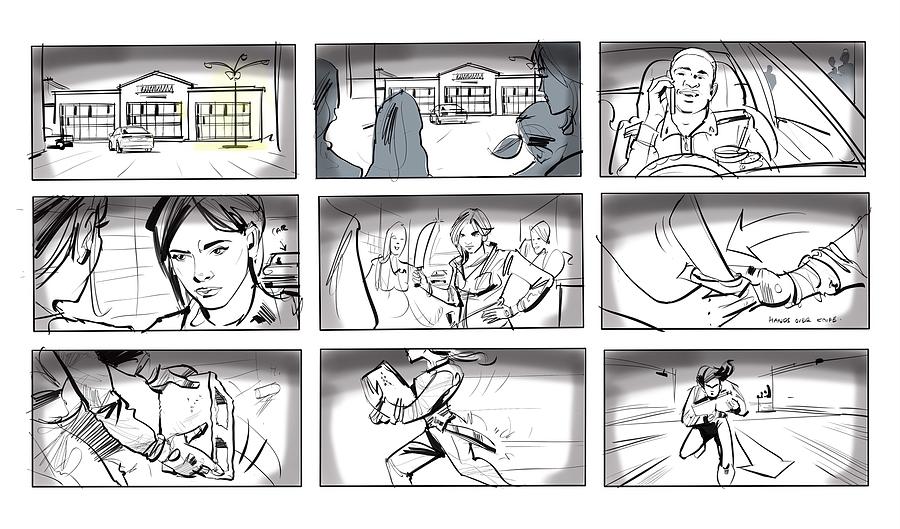This black and white illustration, with faint yellow highlights in the top left cell, is composed of nine meticulously drawn panels arranged in a 3x3 grid. The narrative begins in the top left with a scene featuring a rectangular building with a sloped roof, a faintly illuminated streetlight, and a street where a car is turning left. Nearby, four dark silhouettes are watching the unfolding events. In the adjacent panels, we see a man in a car, holding a drink with a straw and talking on a cell phone.

Transitioning to the middle row, the focus shifts to a woman with an angry expression confronting another woman. Next, this same woman brandishes a machete, with two other women standing menacingly behind her. The following panel depicts an arm holding the machete being handed over to someone else.

In the bottom row, the narrative intensifies as a figure, only identifiable by their gloves and visible arms and legs, picks up a cinder block. This character then appears in the center panel, with a machete attached to their belt, running swiftly to the left while carrying the cinder block. The final panel presents a head-on view of the figure, emphasizing their hurried motion toward the viewer with numerous lines and an arrow pointing forward, signifying speed and urgency.